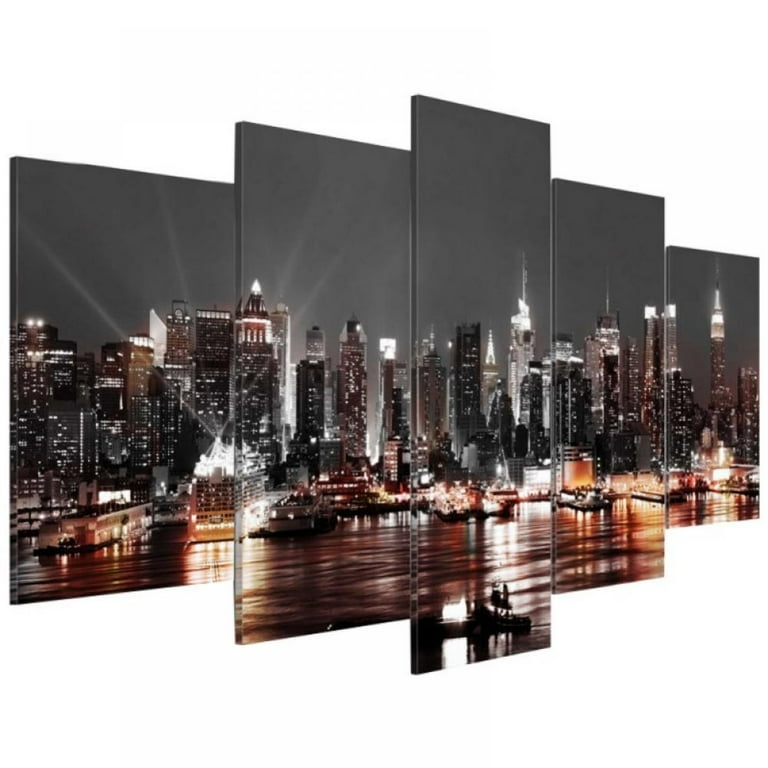A stunning composite image, crafted from five distinct paintings or photographs seamlessly merged to form a cohesive night-time cityscape. The scene is dominated by a sprawling metropolis adorned with towering, illuminated skyscrapers. In the foreground, shorter buildings give way to an expansive body of water, its surface shimmering with reflections of the city's vibrant lights.

A dock extends into the water, where the silhouettes of two individuals stand out, accentuated by the soft glow of a nearby white light. The sky above the city is a moody grayish-black, pierced by dramatic beams of light projecting upwards, creating a striking contrast. The entire composition captures the serene yet dynamic essence of a bustling urban night, enveloped in a mesmerizing interplay of light and shadow.